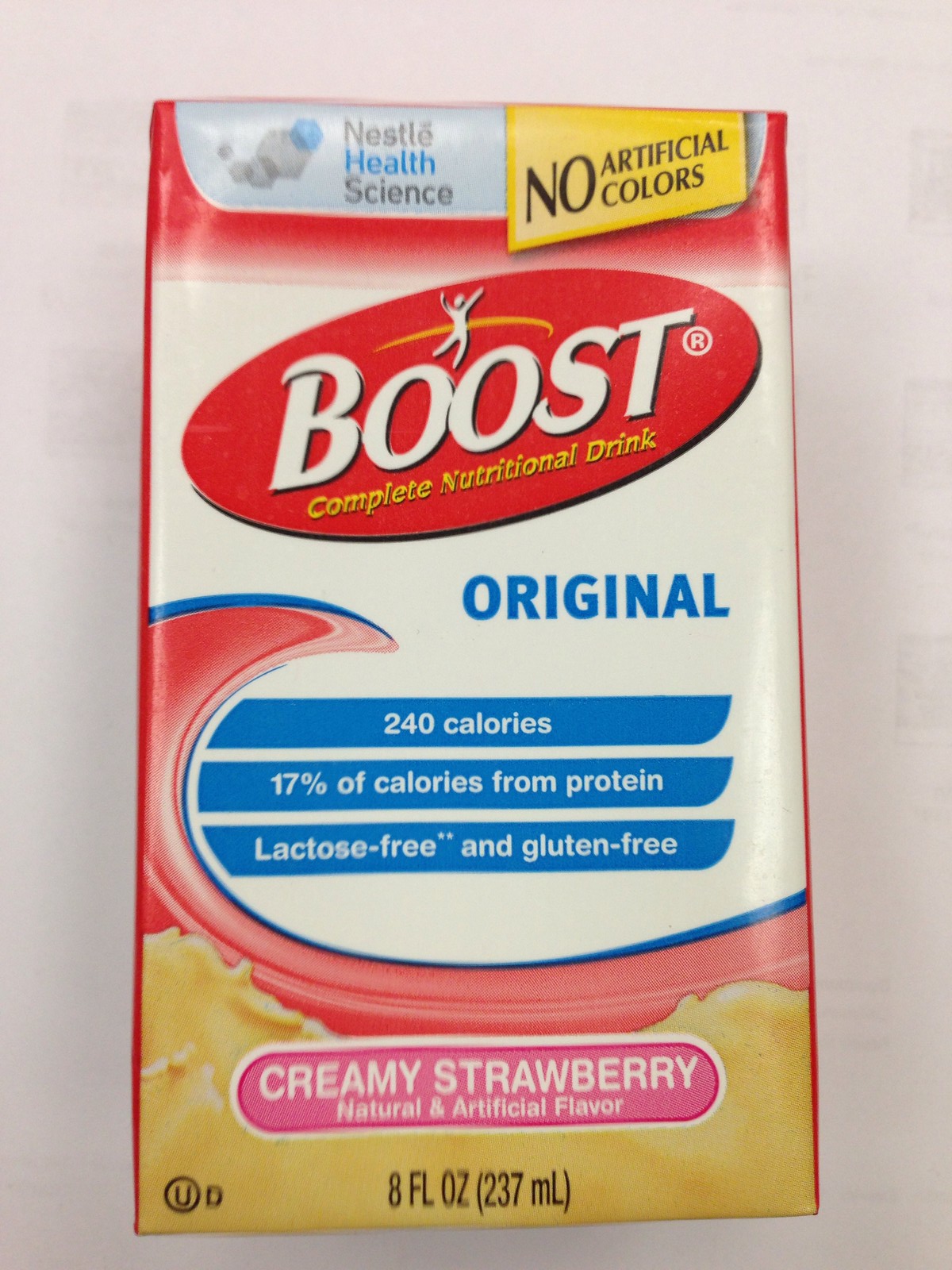The image showcases a rectangular package centered against an off-white background, captured in an up-close view. The top portion of the package features a red background with a white and blue section that has "Nestle Blue Health" written in black, with "Science" beneath it also in black. In the upper right-hand corner, a yellow square bears the text "NO" in large black letters followed by "Artificial" and "Colors" below, both also in black text.

Prominently displayed in the center is a slightly tilted white oval with "Boost" written in bold white letters. Directly below the oval, in blue capital letters, it says "Original." Under this, there are three blue rectangles with white text: the first reads "240 calories," the second states "17% of calories from protein," and the third indicates "Lactose-Free and Gluten-Free." Beneath these rectangles, a reddish-orange wave pattern edged in blue rises on the left side of the package.

The bottom section of the package is yellow, with its top edge forming a wavy line. Centrally positioned within this yellow area is a pink oval outlined in white, containing the words "Creamy Strawberry" in white text.